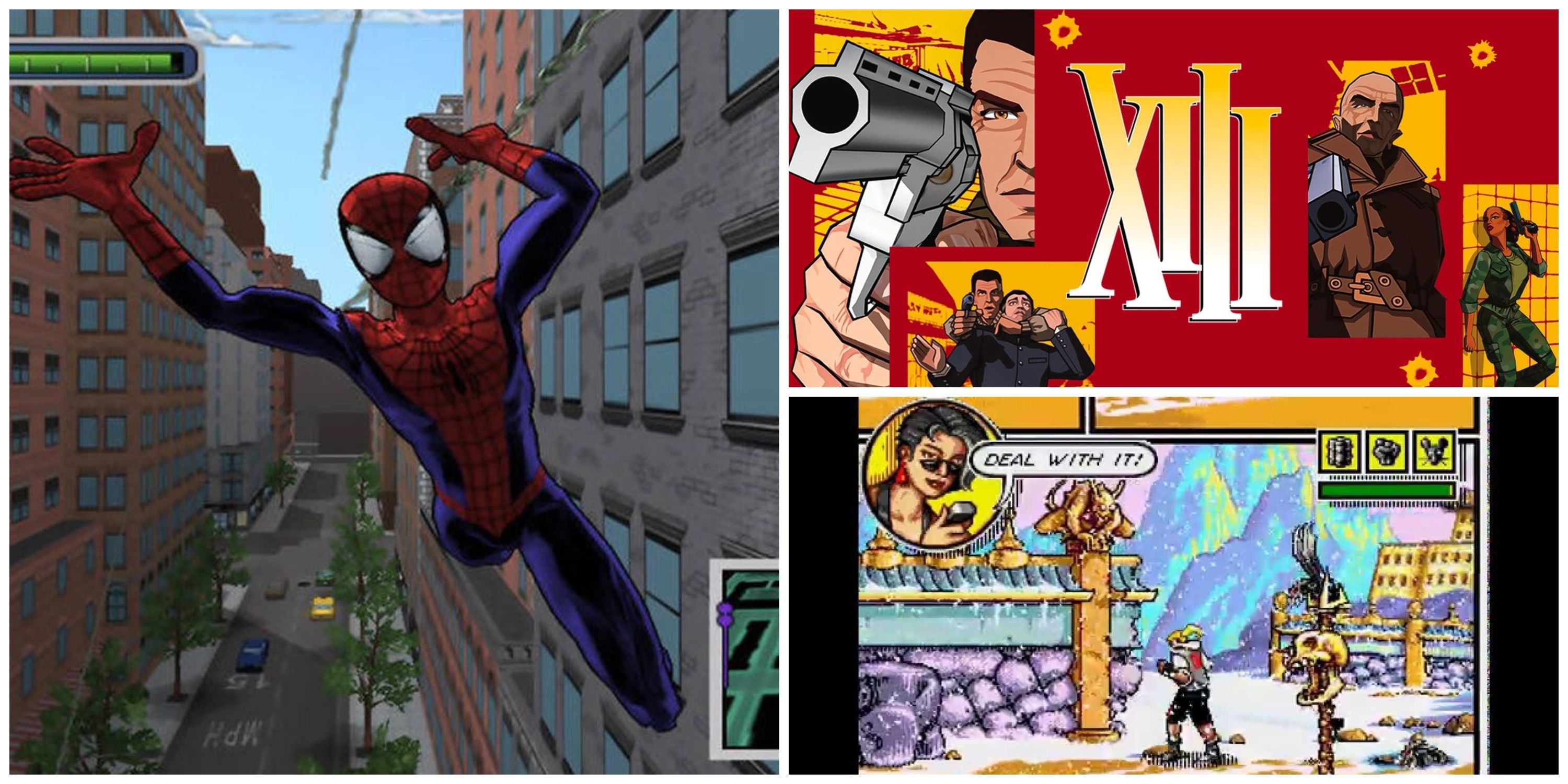This composite image resembles a comic book layout with three distinct sections. On the left, the largest square cell features a vibrant cartoon-style depiction of Spider-Man swinging between two tall buildings colored burgundy and reddish brown. The buildings are detailed with numerous windows, and below Spider-Man, a bustling street scene unfolds with sidewalks lined with trees and cars parked along the road.

The top right cell, set against a red and yellow background, resembles a scene from a shooter video game or comic. It showcases a tense standoff with multiple characters: a man in the foreground brandishes a silver gun, appearing to take another man hostage. On the right, a bald man in a brown coat and a woman in army fatigues, both holding guns, confront the situation. The bold lettering "XIII" is prominently displayed in the center, suggesting the influence of Roman numerals.

The bottom right cell contains a dynamic cartoon-like illustration of a woman with short black hair wearing sunglasses, set inside a circular frame. Emphasizing a defiant attitude, the text "deal with it" accompanies her figure. This image hints at video game elements with its vibrant colors and includes a health bar, reminiscent of a retro fighting game. The background features striking, colorful mountains, completing the collage with a playful yet intense palette.